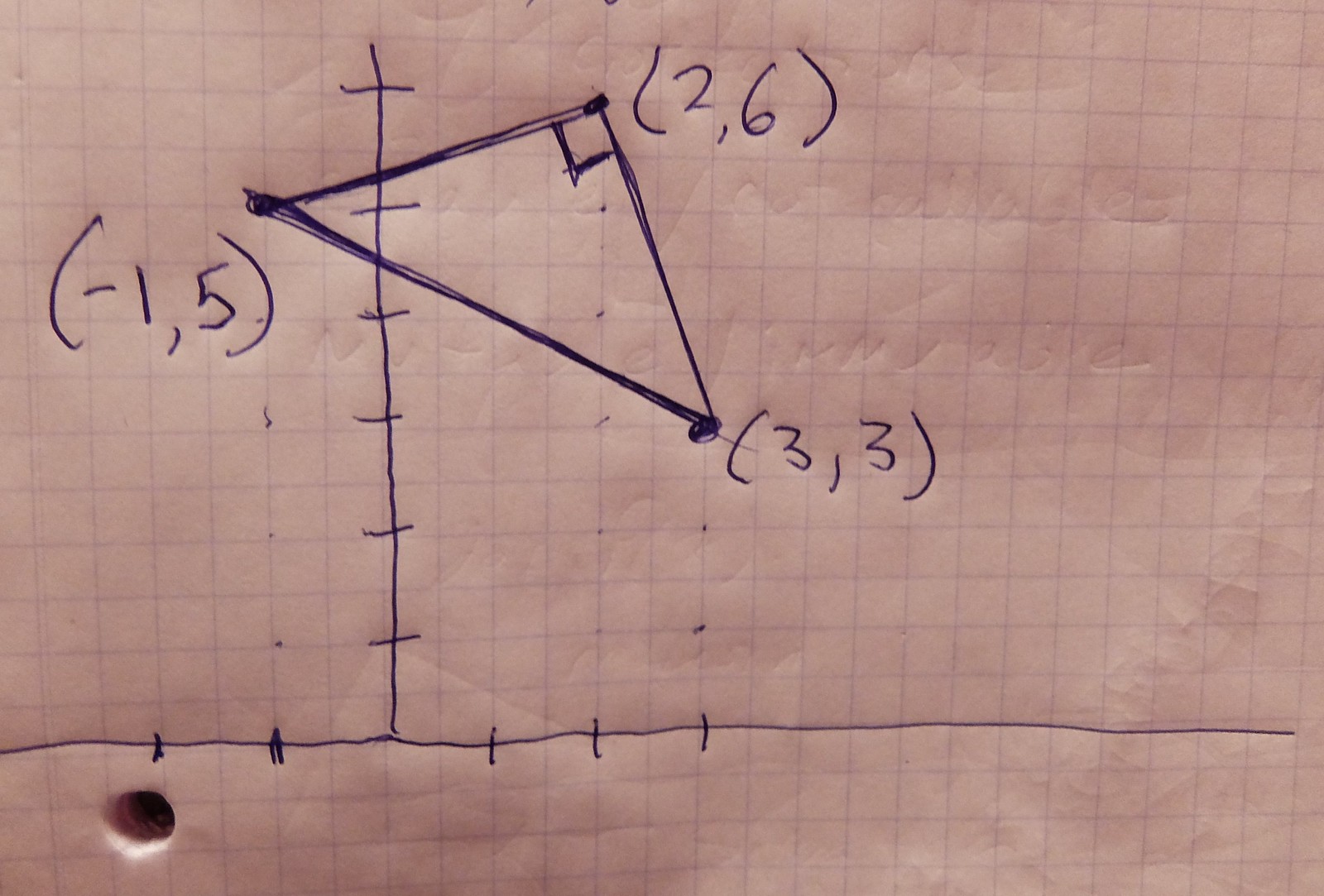This image depicts a photograph of a gridded sheet of paper, taken in an indoor setting. The paper exhibits an extensive array of square grids, upon which numerous handwritten numbers, lines, and shapes are meticulously drawn with a pen. Central to the composition is a T-shaped graph, prominently featuring an isosceles triangle positioned at its top section. The triangle's vertices are annotated with coordinates: (-1, 5) at one corner, (3, 3) at the second corner, and (2, 6) at the top corner. Intriguingly, a small square is inscribed within the top vertex of the triangle. The entire depiction is encapsulated within a rectangular frame, emphasizing the intricate details of the hand-drawn cartography.